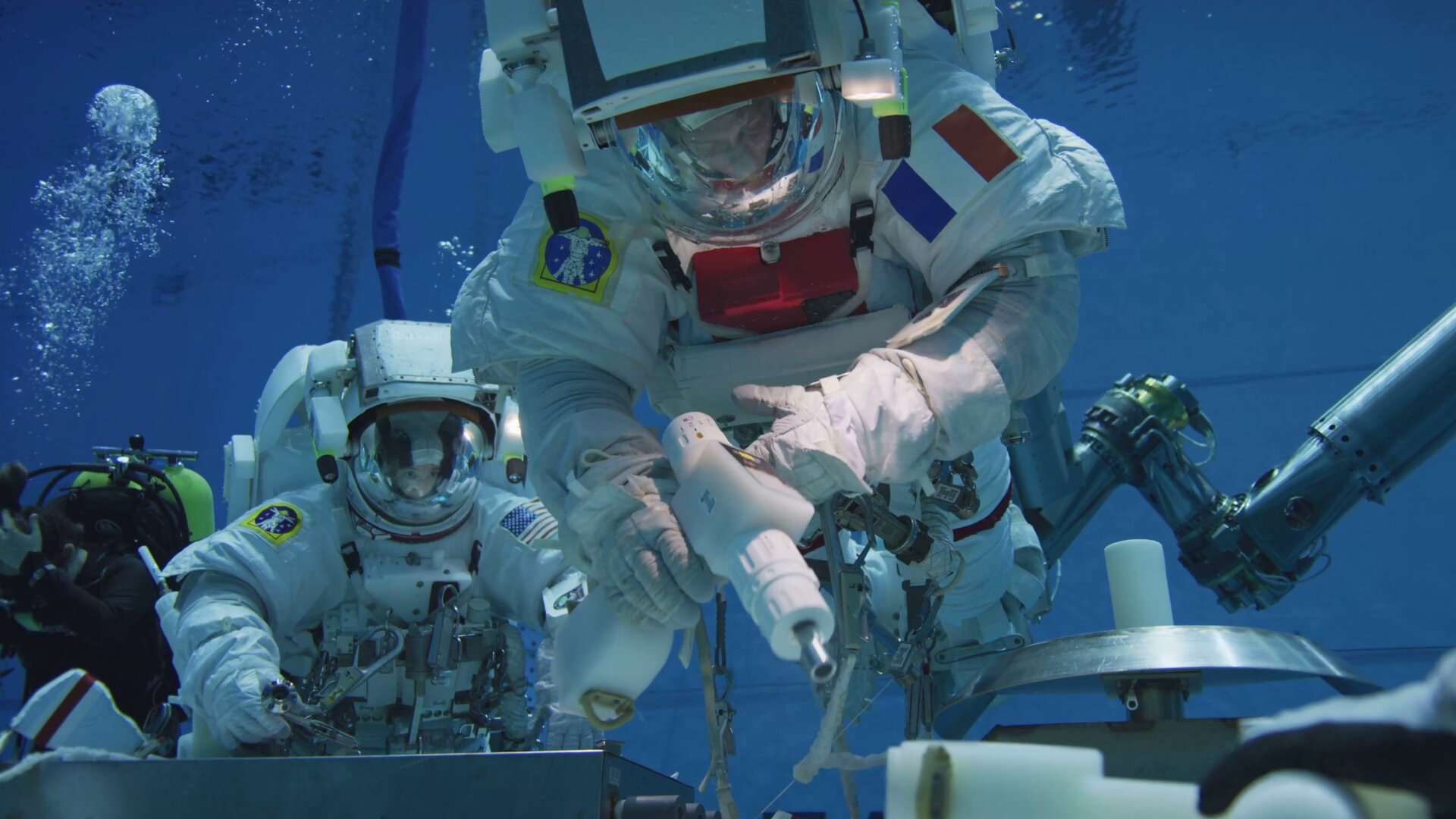This image captures a detailed scene of astronaut training conducted underwater. At the center, two astronauts are immersed in a large pool, wearing bulky spacesuits designed to simulate the conditions of a spacewalk. They are practicing using specialized tools and equipment, one of them holding a drill-like apparatus in his right hand, while the other appears to assist, equipped with a tool belt on his chest for easy access to additional instruments. Both astronauts are connected to the surface by air hoses.

In the background, a diver in standard scuba gear, identifiable by the air bubbles drifting upward, stands by to offer support and ensure safety. To the right of the astronauts, a robotic arm extends into the frame, adding to the realistic simulation of space operations. The surroundings are bathed in a blue hue, possibly from the pool's lighting or painted walls, contributing to the otherworldly ambiance of the underwater setting. At the bottom right of the foreground, a silver cylindrical disc can be seen, possibly part of the training equipment. This alludes to the meticulous preparation these astronauts undergo to master operating in space.